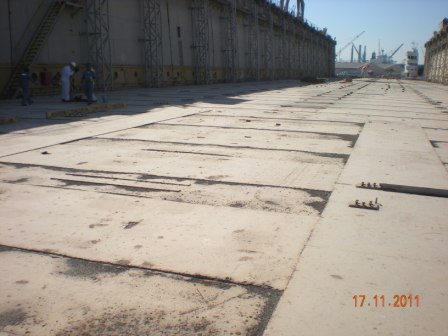In this outdoor photograph taken on 17.11.2011, we are positioned at the edge of a pathway leading toward a bustling pier or harbor, capturing an industrial scene under a clear blue sky. The foreground showcases a deck of worn, light beige steel plates speckled with gray areas and dirt, with some vegetation peeking through the seams. To the left, a darkened wall cloaked in shadow contrasts starkly with the sunlight, revealing outlines of scaffoldings and railings extending along its length. In the upper left corner, three men, partially obscured and difficult to distinguish due to shadows, appear to be working near a ladder or steps leading up from the floor. One of the men is clad in white clothing, including a hat. To the right, a gray wall extends toward the horizon, beyond which towers, an overhead crane, and a ship are visible, hinting at the port's busy activity. This image is marked with a red date in the bottom right corner, marking it as taken on 17.11.2011.